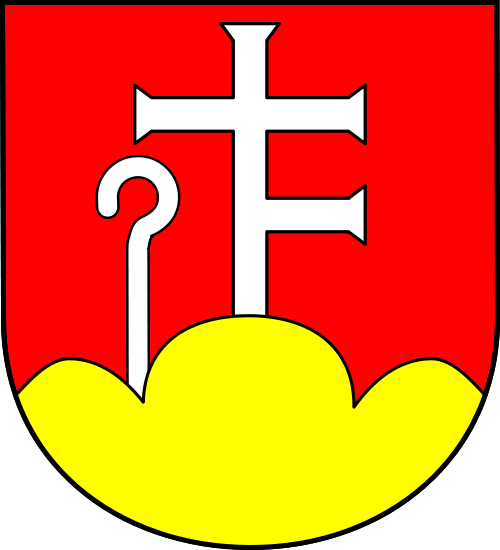The image depicts a simple shield with a distinctive black outline. The shield has a straight top edge and sides that curve inward three-quarters of the way down, eventually forming a perfect semicircular bottom. The background is divided into two sections: a larger red field occupying the top area and a smaller yellow section resembling a cloud with three bumps, the largest bump in the middle, just above the base.

Central to the red background is a complex white emblem. A vertical bar rises from the yellow cloud-like base, topped with a funnel-shaped flange. This bar is intersected by a crossbar that extends horizontally with similar flanges at both ends. Additionally, lower down, a shorter arm with the same funnel-shaped flange aligns with the central bar. To the left of this structure is a shepherd’s hook-like figure that curls to the left, resembling a question mark with an extended leg.

Overall, the image combines elements of heraldic and possibly symbolic nature, featuring a detailed, multicolored background and intricate white emblems set against a strikingly bold outline.